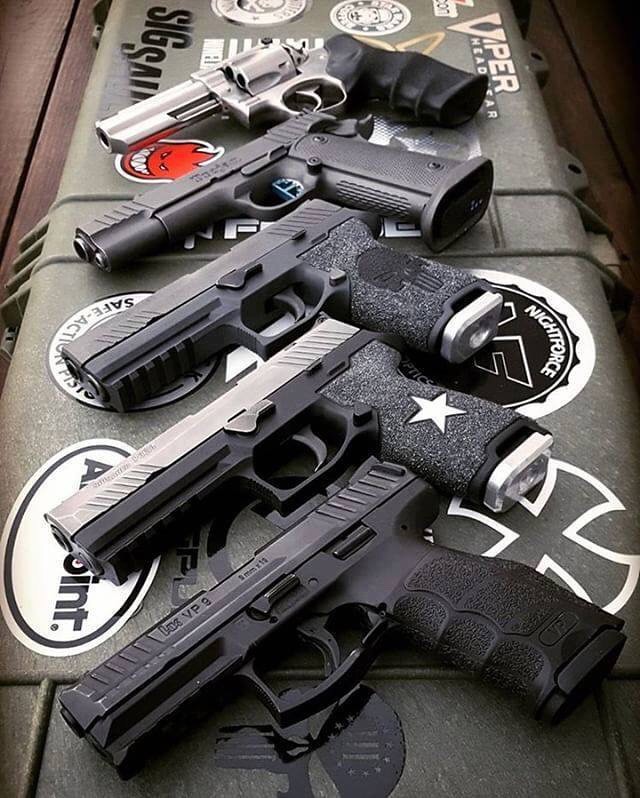In this photograph, which is in portrait orientation, we see a detailed display of five handguns organized on a rectangular, black gun case adorned with various stickers. The brightly lit image highlights the nature of each firearm. The guns are arranged horizontally with their handles to the right and barrels to the left, and they exhibit a range of designs and colors though they predominantly feature dark tones with some silver elements.

The first handgun is entirely black with a matching handle, while the second one includes a silver top and a white star on its gray speckled grip, connected to a black lower part. The third pistol has a gray and silver bottom with a white speckled handle and a black top. The fourth gun is all black, save for its silver trigger. The fifth and last firearm, which stands out with an emphasized barrel, has a black grip and a silver body, featuring a cylindrical part for loading bullets. 

All of these handguns are laid out on a rugged, military-green gun storage container, which is decorated with several eye-catching stickers, including a red grinning evil face, and the word "Viper" visible at a distance, along with a cross towards the front. The storage surface further emphasizes the context and nature of this detailed display.